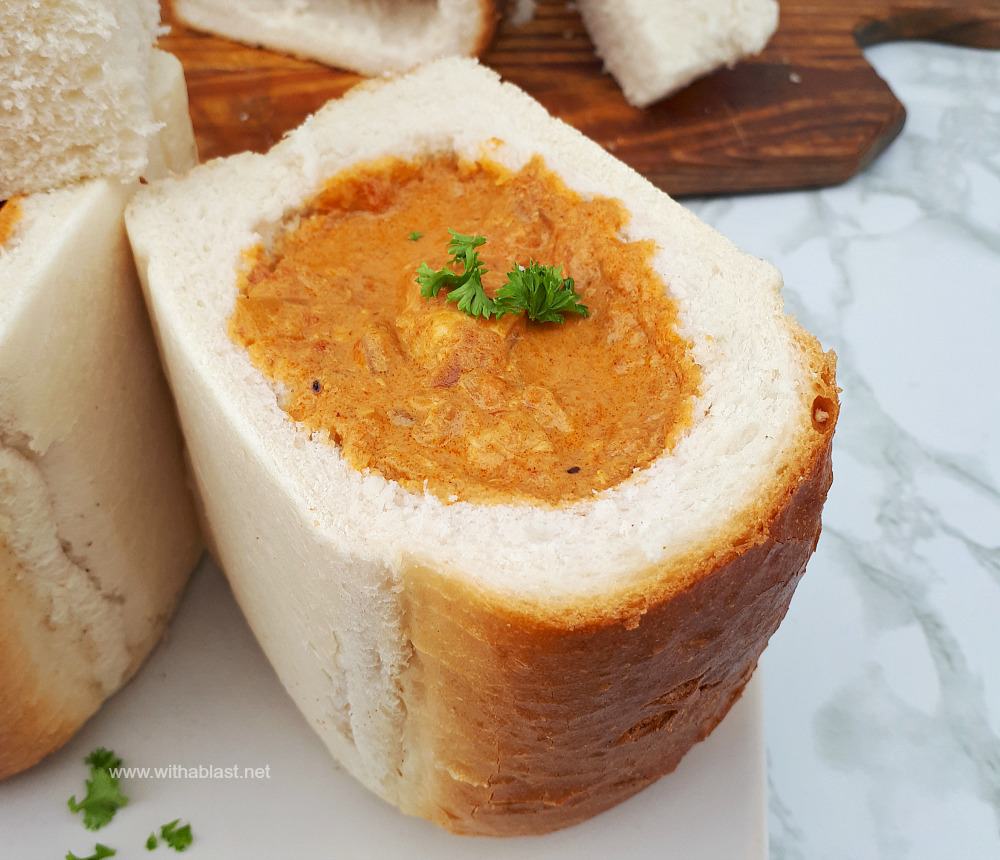In this detailed photograph, we see a culinary creation consisting of a hollowed-out loaf of bread filled with a thick, orange-colored paste or soup, which bears a resemblance to peanut butter. The bread is a distinctive white loaf with a golden-brown crust, a result of being baked to perfection. A generous portion of the filling is visible, as an end of the loaf has been sliced off, exposing the rich, creamy interior.

The bread is elegantly presented on a pristine white plate that rests on a polished granite marble countertop. In the background, a portion of a wooden cutting board with additional slices of bread can be seen, indicating ongoing preparation. The sliced bread scattered nearby suggests that perhaps more servings are being readied, possibly to be filled with the same savory stuffing. 

As a final touch, the filling is garnished with a few fresh parsley leaves, adding a pop of green that contrasts beautifully with the warm, orange hue of the stuffing. The overall setting, with the clean white plate and sophisticated countertop, frames this dish as both traditional and gourmet, inviting curiosity about the exact nature of the filling and its origins.